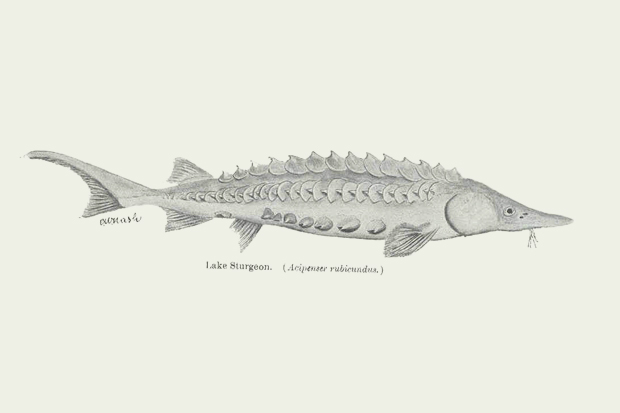This detailed illustration showcases a Lake Sturgeon, as identified by the text "Lake Sturgeon" followed by its Latin name in parentheses below the image. The drawing is rendered in a pencil-gray color, presenting the fish in a free-floating silhouette with a focus solely on its exterior. The Lake Sturgeon has a long, slender body with a distinctively tapered, flattened snout and a single visible eye. 

Notably, the sturgeon appears heavily armored, with its back and sides adorned with sharp, protruding spikes or scaly plates. These unique features give the sturgeon an almost menacing appearance. The fish’s body is equipped with multiple fins—two smaller ones along the sides and additional fins positioned towards the chest area. The tail fin is particularly interesting, shaped somewhat like a bottle opener, emphasizing the fish's streamlined form.

The sturgeon's underbelly appears rugged, almost as if it has rocks protruding from it, adding to the armored and somewhat ferocious visage of the fish. Detailing on the tail fin includes visible striations. The entire depiction, clean and without a specific background, conveys the essence of this ancient and formidable freshwater species.